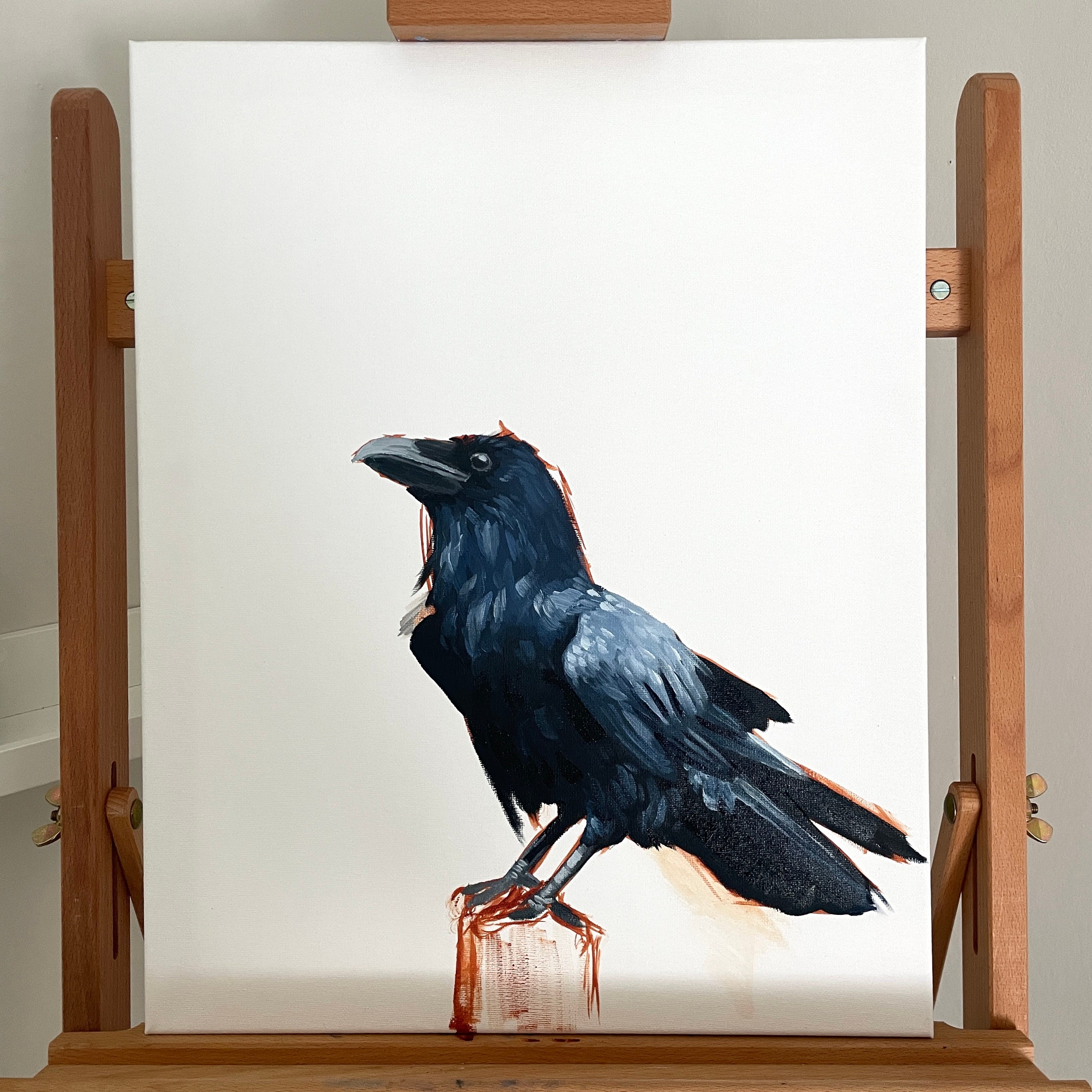The image features a detailed painting of a crow displayed on a wooden easel. The crow, painted in shades of black and lighter silver, shows off its distinctive thick beak, stubby tail, and intricate feathers that create a silver sheen. The canvas is stark white, making the crow stand out vividly. The bird takes up roughly the bottom half of the canvas, perched on an earth-like surface which is partly obscured and somewhat ambiguous. There is a striking detail of red around its tail feathers and talons, with a smudged appearance that might suggest blood, adding a dramatic touch to the painting. The crow's eye is painted in a way that seems to gaze directly at the viewer, imparting a realistic and intense look. The overall painting is very detailed, highlighting the artist’s skill.